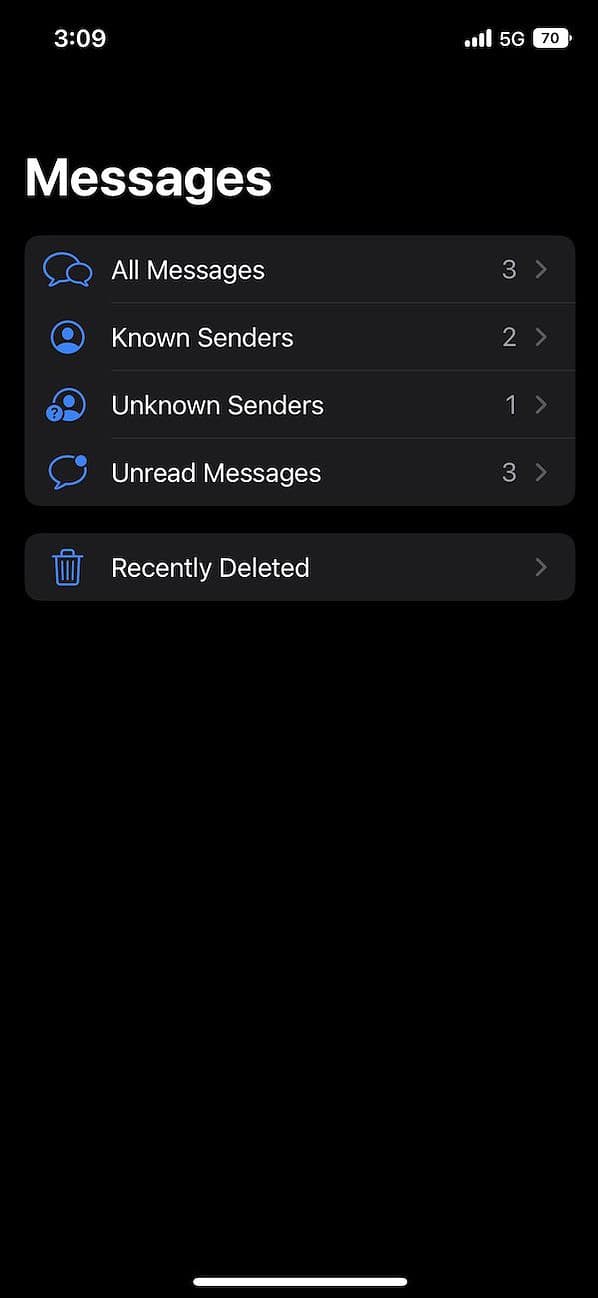This image is a screenshot of an iPhone Messages app interface. 

- **Status Bar**: 
  - At the top left corner, the time is displayed as "3:09" in white text.
  - The service signal bars are full, indicating strong reception.
  - The network is connected to "5G."
  - The battery icon shows a 70% charge.

- **Background**: 
  - The entire background is black.

- **Header**: 
  - The word "Messages" is prominently displayed in white letters.

- **Sections**:
  - **All Messages**:
    - Icon: Two blue speech bubbles.
    - Label: "All Messages" written next to the icon.
    - Indicator: A "3" is shown on the far right with a right-facing arrow indicating navigation to the messages.
  
  - **Known Senders**:
    - Icon: A blue circle with a person's silhouette inside.
    - Label: "Known Senders" in white letters to the right of the icon.
    - Indicator: A "2" on the far right with a right-facing arrow.
  
  - **Unknown Senders**:
    - Icon: A circle with a person silhouette and a smaller circle with a question mark overlay.
    - Label: "Unknown Senders" in white letters to the right of the icon.
    - Indicator: A "1" on the far right with a right-facing arrow.

  - **Unread Messages**:
    - Icon: A text bubble with a blue dot inside.
    - Label: "Unread Messages" in white letters.
    - Indicator: A "3" on the far right with a right-facing arrow.
  
  - **Recently Deleted**:
    - Icon: A trashcan symbol.
    - Label: "Recently Deleted" in white letters.
    - Indicator: A right-facing arrow with no number displayed.

- **Swipe Indicator**:
  - A white stripe "swipe-up bar" is visible at the very bottom of the screen.

This screenshot comprehensively displays the various message categories within the iPhone Messages app along with their respective icons and navigation indicators.